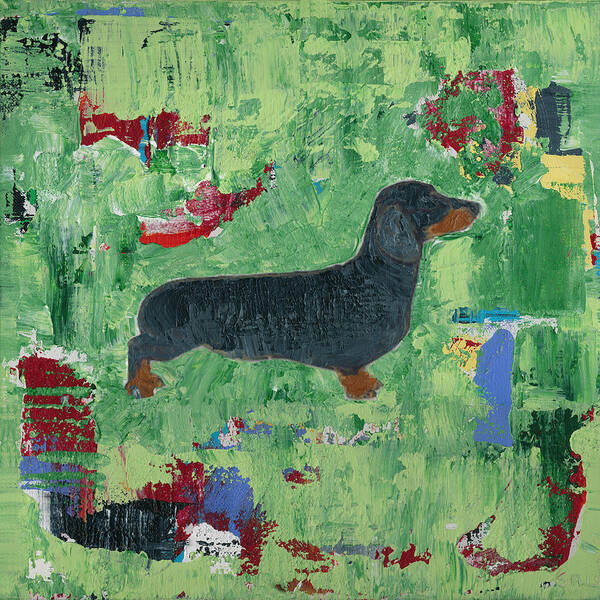The painting features a classic black Dachshund, often referred to as a wiener dog, viewed from the side with its head turned to the right. Its distinguishing features include a black coat with dark brown accents on its muzzle and all four paws. The background of the painting is predominantly green, with a mix of darker greens central to the piece and lighter greens towards the upper and lower edges. The green backdrop is textured with visible, purposeful brush strokes that suggest an uneven, possibly abstract setting. Scattered throughout the background are vibrant splotches and strokes of red, light blue, white, and black paint, concentrating more on the lower left-hand side and with a noticeable splash of yellow in the top right corner. The use of multiple layers of acrylic paint gives the impression of a rich, layered artwork, possibly hinting at an underlying complexity or previous layers similar to graffiti. The overall feel is one of a vivid, dynamic setting serving as a backdrop to the prominently detailed Dachshund.